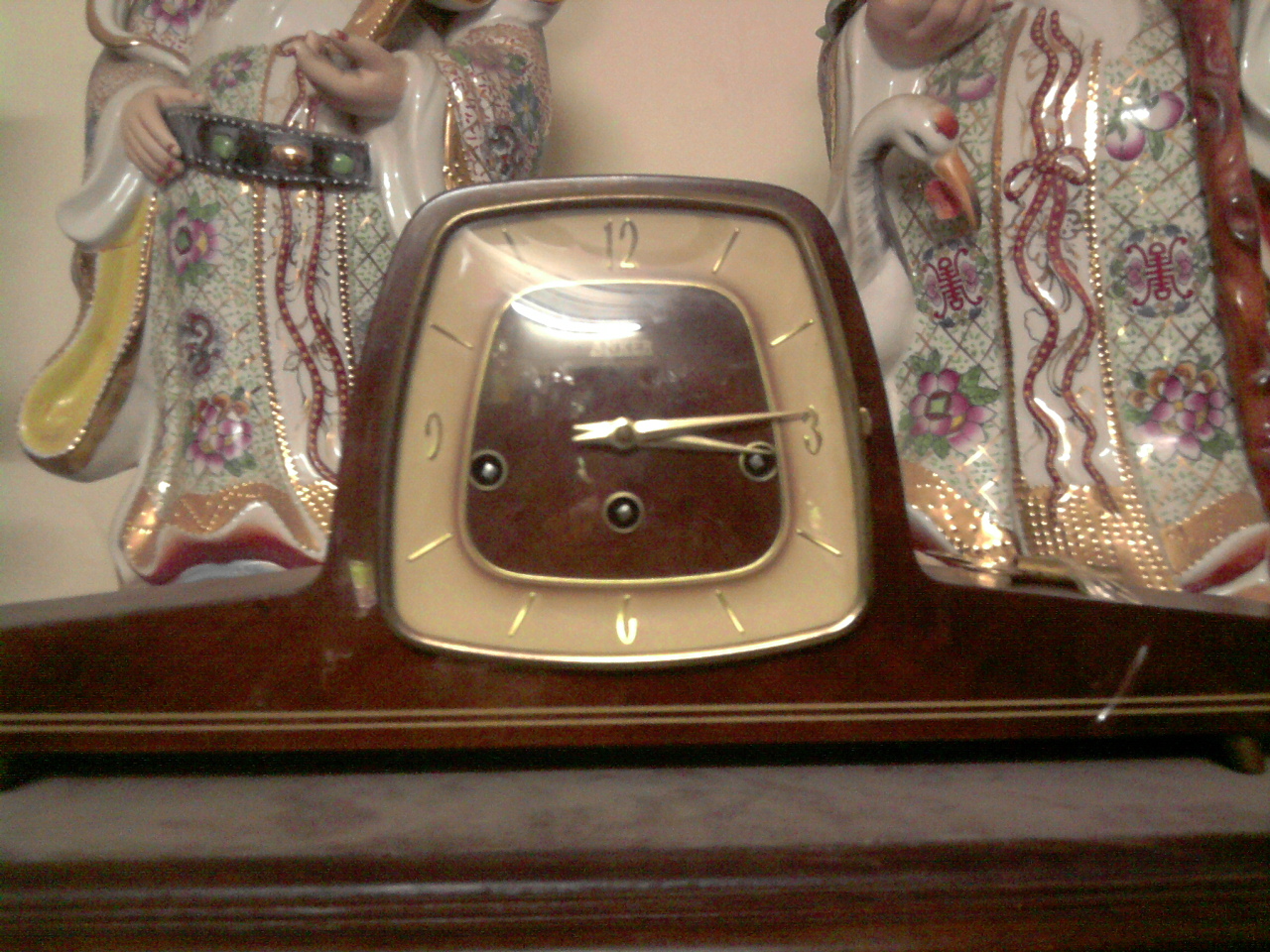The image captures an intricate interior scene, dominated by detailed statues and a central clock. Elevated atop a structure, a ceramic statue catches the eye. It holds a black belt adorned with white dots in one hand and features green and red gem embellishments. The statue's other hand is outstretched, with both arms depicted as if wrapped in rope, exhibiting patterns of red ropes descending from its left side. Floral designs embellish the backdrop, creating a green grid effect. To the right, the scene is accentuated by another ceramic statue of a stork, poised as if gazing over a bridge.

In the center of this tableau, a vintage clock face claims attention. Displaying the numbers one through twelve, with three, six, nine, and twelve standing out, the clock's brown face is marked with dash lines and houses three winding dots. The minute hand points precisely at three, while the hour hand rests between three and four. A brand logo, reflected by ambient light, adds a touch of authenticity. The entire composition is set atop a countertop, blending artistry and timekeeping in a harmonious interior display.